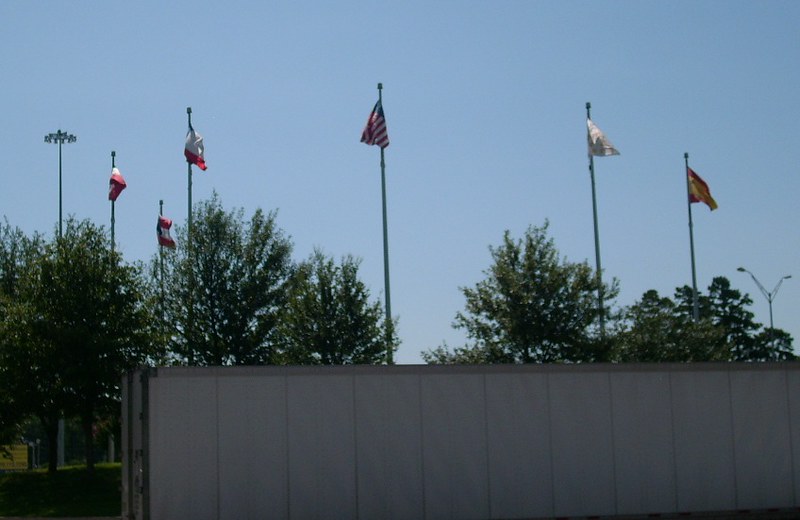This photograph, taken outdoors, captures a scene with a hazy blue sky as the backdrop. Dominating the upper portion of the image are six flagpoles, with flags fluttering in the wind. The central flagpole prominently displays the American flag. The flags on either side are partially visible; the three on the left feature red and white colors, one resembling the Texas flag with a single blue star, while the ones on the right exhibit a mix of white, gray, red, and yellow hues. Below the flagpoles, a tree line with five trees, sporting dark green leaves, partially obscures the view. At the very bottom, a long, gray, rectangular storage container stretches from the bottom right to the bottom left. Flanking the scene, light poles are positioned on both the left and right sides, enhancing the outdoor setting.